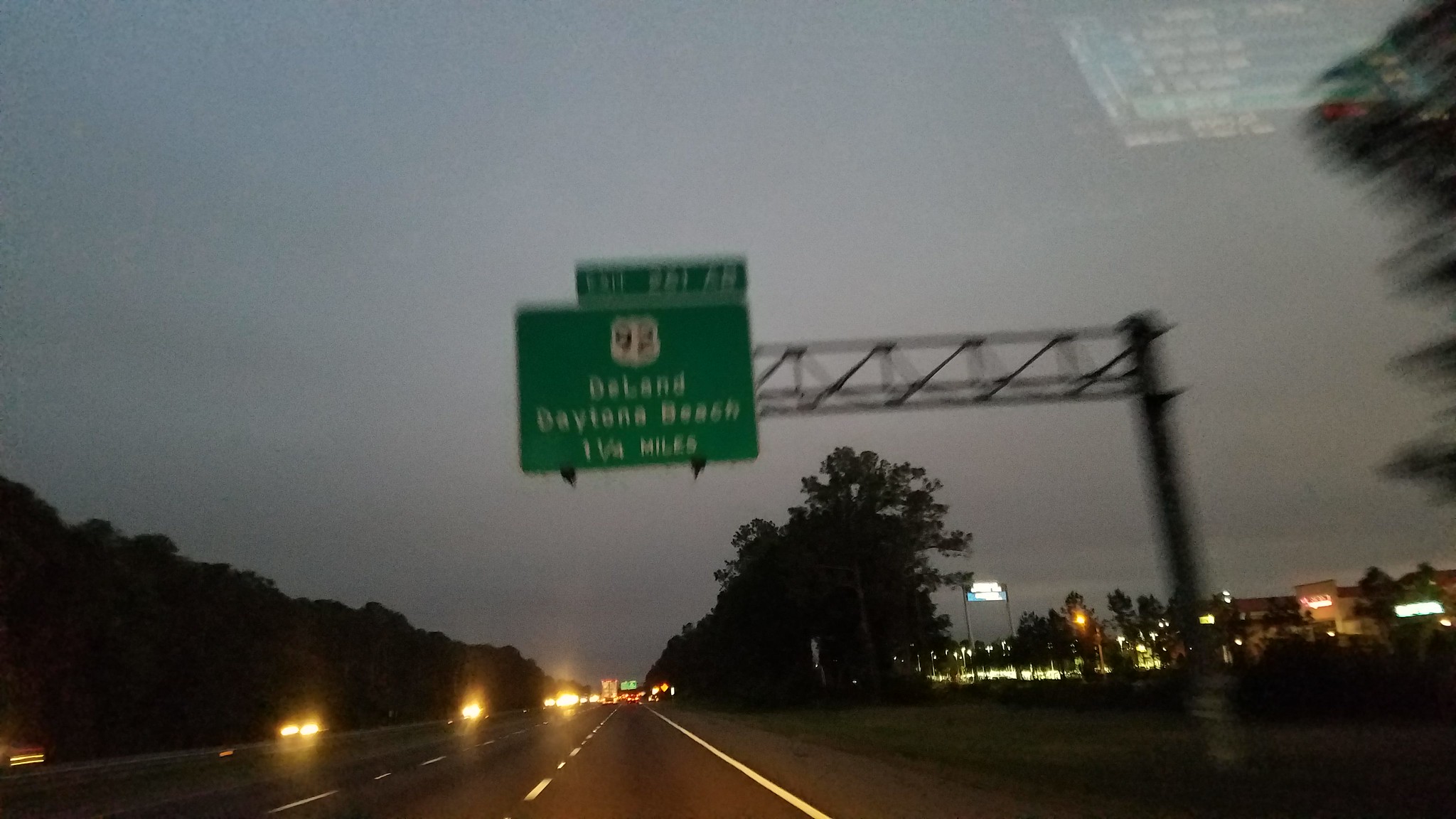In this nighttime photograph, we are peering down a large highway, captured from within a car, evidenced by a slight reflection on the window. The image, though slightly out of focus, reveals a vast, empty stretch of road devoid of discernible vehicles. Suspended above the highway is a green exit sign displaying "Exit 221" in bold white letters. Adjacent to this, a smaller white sign distinctly marks "92." Below these indicators, additional text directs travelers to "DeLand, Daytona Beach," with a distance marking of approximately one and a half miles. On the right side of the highway, a building, likely a hotel, is faintly visible, while leafy trees line both sides of the road, adding a touch of greenery to the nocturnal scene.